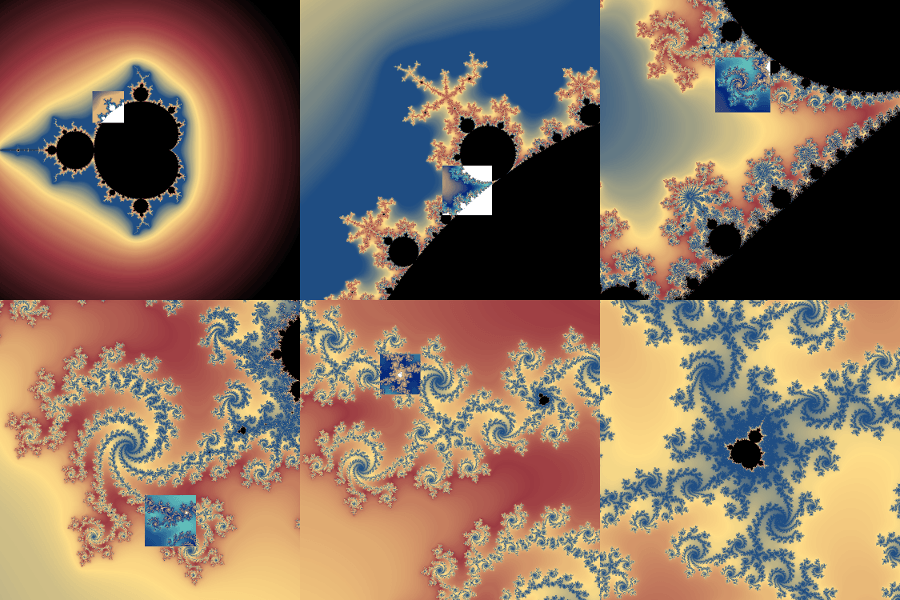The image is a vivid and intricate collage of six panels, each depicting a close-up, fractal-like pattern that repeats infinitely. At the heart of the design is a central black area with a heart-like shape topped by a circle, surrounded by successive outlines of yellow, blue, blurrier yellow, and red hues, all set against a black canvas. Dominated by a palette of oranges, yellows, reds, and blues, the images evoke a sense of floating, almost cellular structures, with swirls and branching patterns that vary across panels. Scattered black dots accentuate the intricate geometrical formations, creating a unique, almost otherworldly aesthetic. While the patterns are asymmetrical and random, they collectively suggest a deep, scientific or cosmic examination, unfolding an endless zoom into the fractal-like artwork.